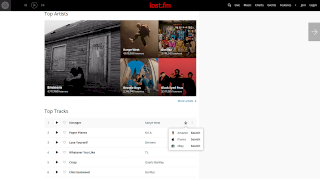The web page has a clean white background with a prominent black bar running horizontally across the top. In the center of this bar, "last.fm" is written in bold red letters. On the upper right side of the bar, there are several web links displayed in white text. Additionally, a white arrow set against a gray background, pointing to the right, is positioned at the top right of the image.

In the middle section of the web page, there is a collection of five images. The leftmost image is monochromatic, featuring shades of gray, white, and black. To the right of this image is a quadrant of four colorful images arranged in a square. The lower right image within this quadrant shows a dark pink or reddish background with three men standing side by side, all dressed in black attire.